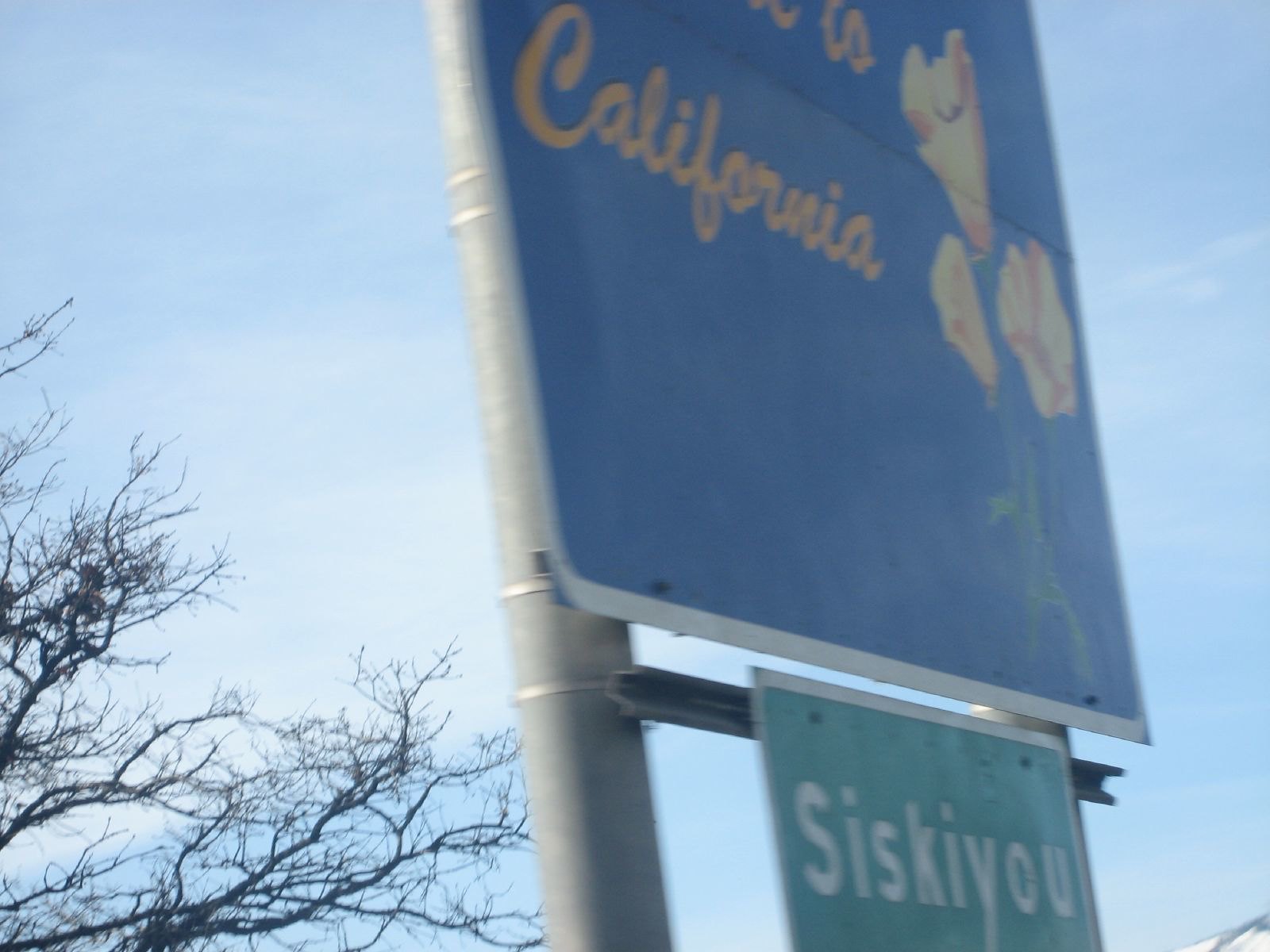Against a backdrop of a brilliant blue sky dotted with wispy white clouds, a striking scene unfolds. In the lower-left corner, stark black tree branches, stripped of their leaves, frame the image with a dramatic touch. Dominating the center, a prominent sign affixed to a silver metal pole captures attention. The upper portion of the sign is a vibrant blue, elegantly featuring the word "California" in cursive. To the right of this text, an artistic flourish of yellow and orange flowers with slender green stems adds a splash of color. Just below, a second sign in green, bordered in white, reads "Siskiyou" in bold letters. This green sign is supported by a black bar spanning beneath the blue sign, completing the structured yet picturesque composition.